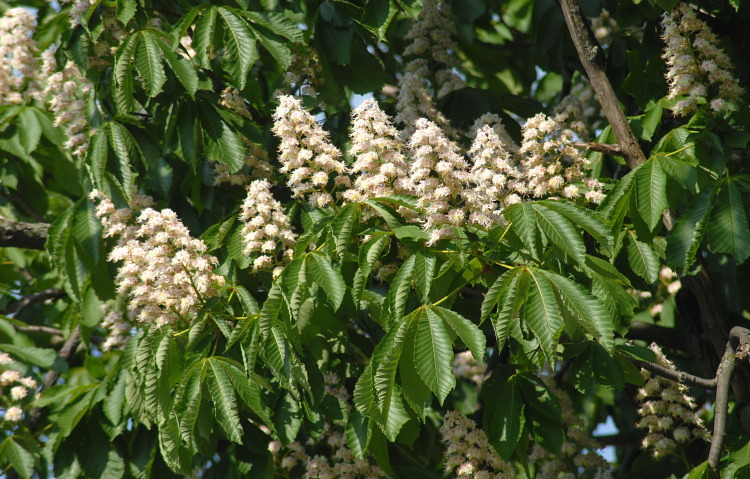The image captures a close-up of a nature scene featuring a cluster of white, cone-shaped flowers and green leaves. These flowers, resembling small and tall pollen-like structures, are densely packed and positioned atop a bush. The scene is framed by green leaves at the base, which appear as standard foliage growing from the stems. Although it is daytime, possibly early evening, the blue sky in the background is largely obscured by surrounding trees. In the upper left and upper right sections of the image, the white flowers extend and cluster in various directions. A prominent branch is visible on the left side of the photo, extending vertically from the bottom right to the top. The scene captures the lush, layered intricacies of plant life in a serene natural setting.